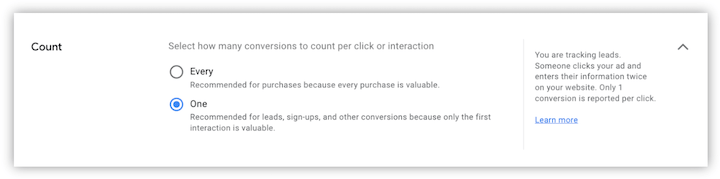This image is a detailed screenshot from a computer programmer's website, showing a user interface for an analytical software tool designed to track and count user interactions and conversions. The interface is encapsulated in a thin white box with a subtle grey shadow bordering its edges. On the left side of the screen, the word "Count" is prominently displayed, followed by a description in the center of the screen, "Select how many conversations to count per click or interaction."

Below this, there are two options within boxes: "Every," which is recommended for purchases ("because every purchase is valuable"), and "One," which is highlighted with a blue checkmark and is recommended for leads, sign-ups, and other conversions ("because only the first interaction is valuable").

On the right side of the screen, a text explains the functionality: "You are tracking leads. Someone clicks your ad and enters their information twice on your website. Only one conversion is reported per click." An upward-pointing arrow follows this text.

Underneath the main content, there is a blue text link labeled "Learn more," suggesting additional information is available. The overall purpose of this interface seems to be for users to configure and understand how their advertisements are tracked for conversions. The interface is clean, straightforward, and designed for ease of use, aimed at those looking to optimize their ad performance without requiring deep technical knowledge.